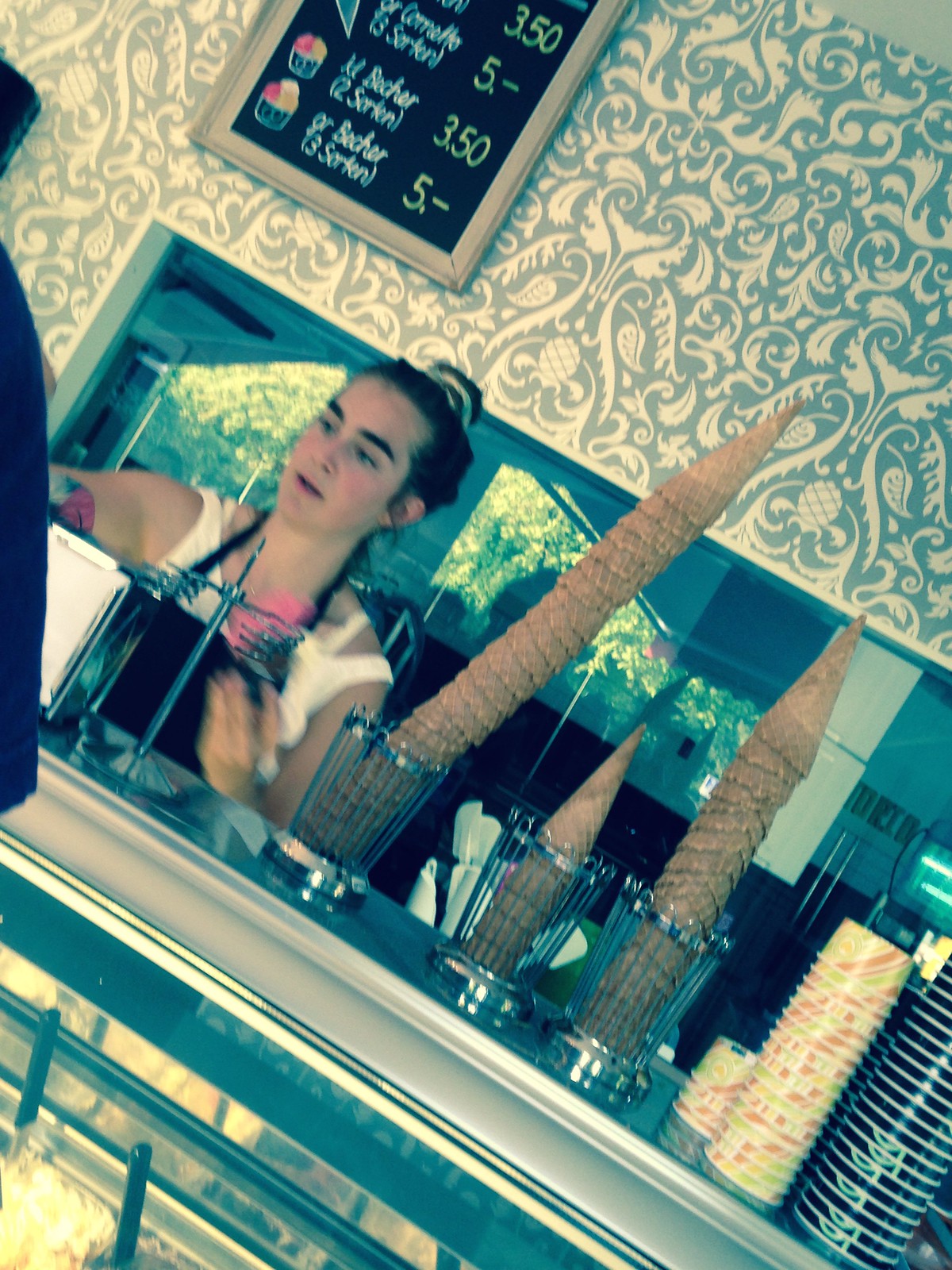In this photo, taken at an ice cream shop, the image is slightly tilted and off-center, capturing a lively and detailed scene. The backdrop features striking blue and cream-colored ornate wallpaper with intricate, unique designs, adding a whimsical charm to the setting. At the center of the image stands a young woman with dark hair pulled up in a bun. She has thick eyebrows and a fair complexion, wearing a white tank top and a black apron, engaged in conversation with a customer while presumably taking an order. 

Behind her, a rectangular chalkboard menu in a wooden frame displays prices, clearly visible are $3.50 and $5, though the specific items aren't discernible. The counter in front of her is adorned with three glasses, each containing a stack of inverted sugar cones, alongside a variety of paper ice cream cups. To the left sit some lighter-colored cups with red and green stripes, and to the right, partly cut off, are larger black cups with white rims. Adding to the functional aspect, a package of napkins lies on the counter, readily accessible for customers. The entire setting is further highlighted by the partial view of a freezer and mirrored surfaces, reflecting the welcoming ambiance of the shop.